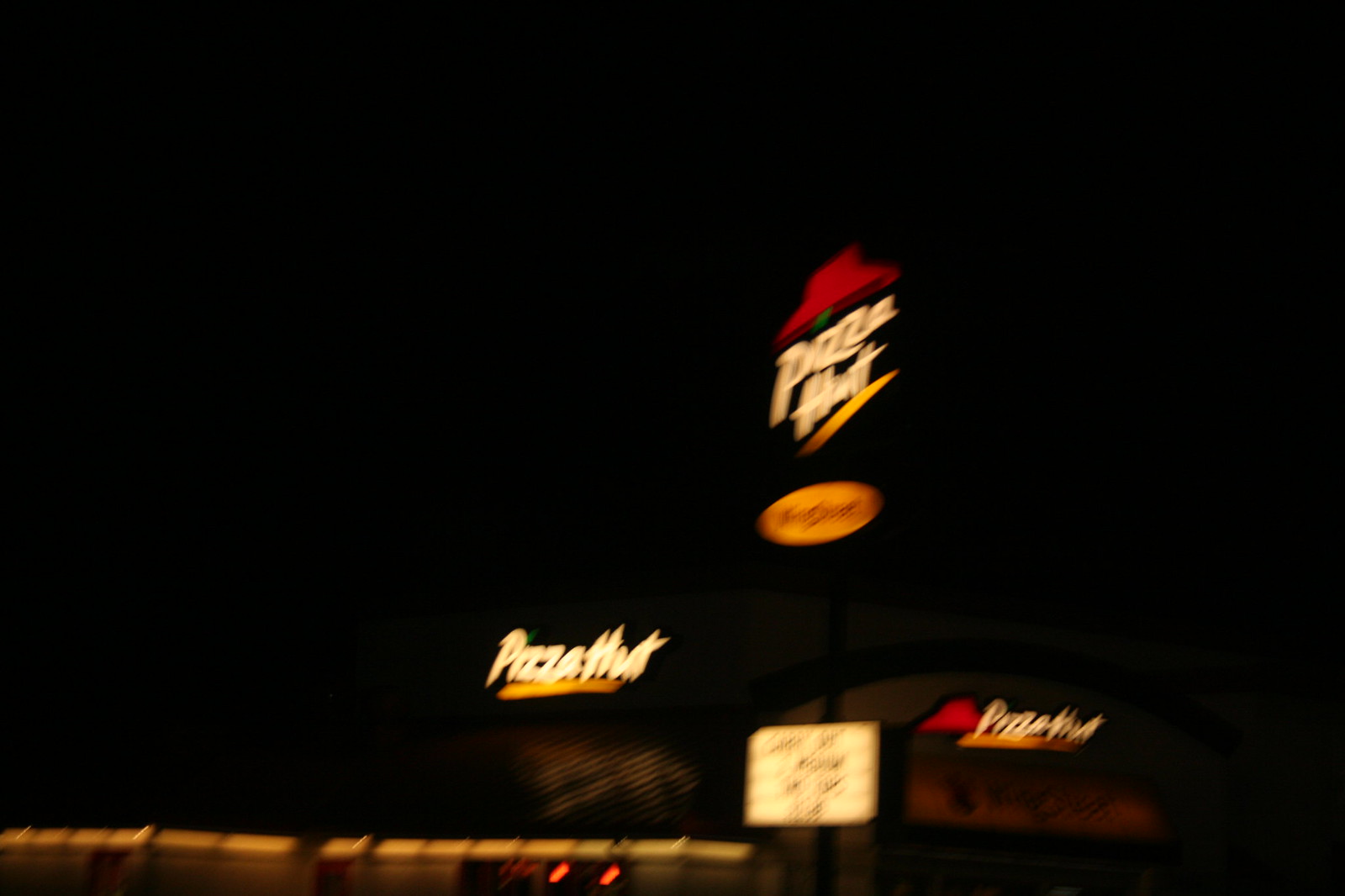The image captures a nighttime scene featuring a very blurry Pizza Hut establishment. Dominating the upper half of the picture is the dark, night sky. In the middle bottom section, white letters spell out "Pizza Hut" with a yellow underline. Directly above, a billboard-like sign also displays "Pizza Hut" in white letters, accompanied by the iconic red roof logo above it. Below this are two more signs; a yellow circular one and a white square one with illegible black text due to the blurriness and distance of the photograph. To the right, another "Pizza Hut" logo appears with a yellow underline, and the red roof logo is positioned to the left of this particular text. The overall impression is a somewhat cluttered arrangement of Pizza Hut branding elements, all captured in a distinctly blurry and distant nighttime shot.